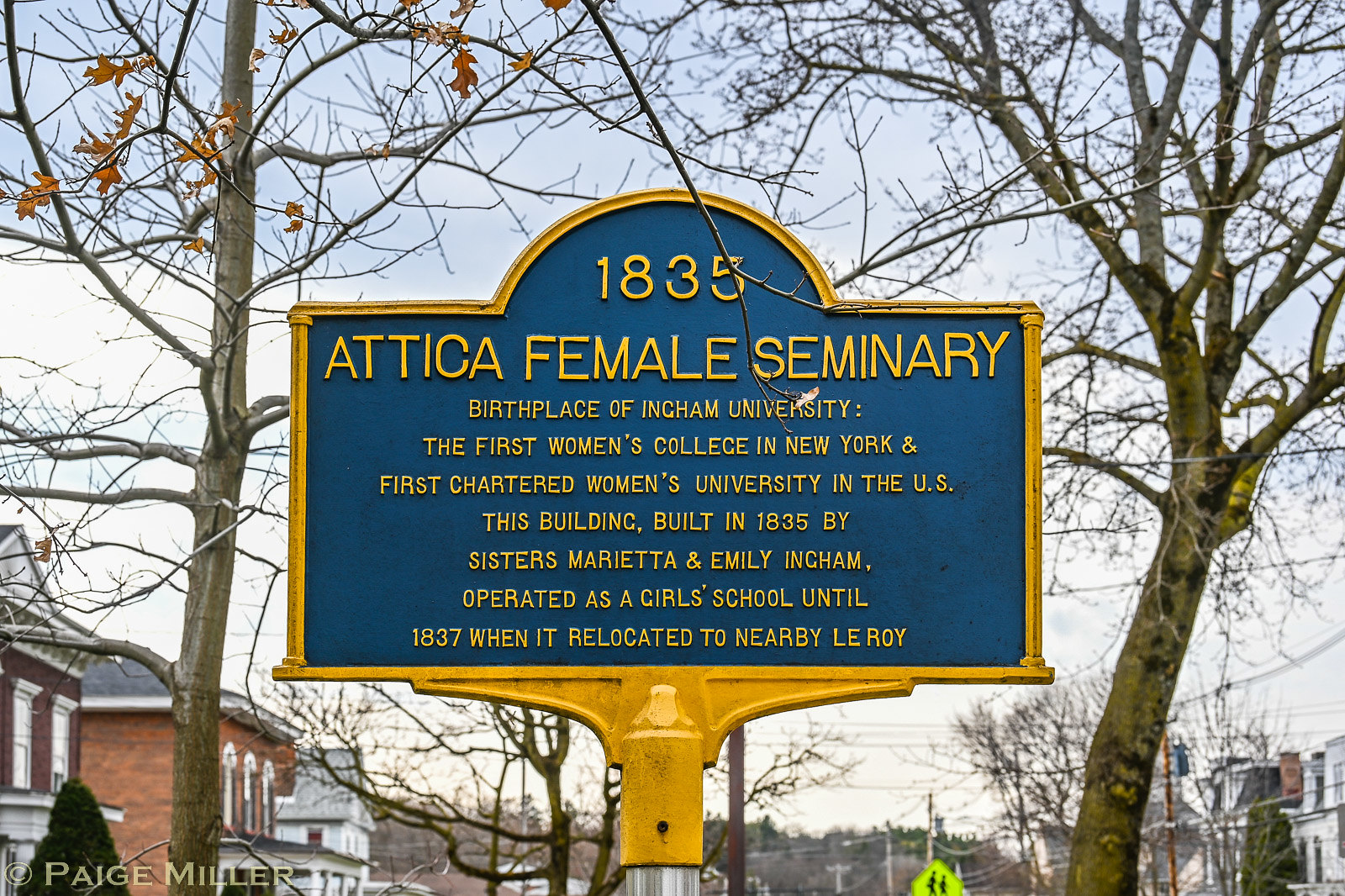The image prominently features a blue and yellow historical sign that reads: "1835 Attica Female Seminary, birthplace of Ingham University, the first women's college in New York, and the first chartered women's university in the U.S. This building, built in 1835 by sisters Marietta and Emily Ingham, operated as a girls' school until 1837, when it relocated to nearby Leroy." The sign has a rich blue background with gold trim and yellow text. In the background, a somewhat bleak sky and sparse, mostly leafless trees suggest winter. A neighborhood with a mix of colonial-style brick buildings and houses can be seen, along with a pedestrian sign near the bottom of the frame. The name "Paige Miller" appears in the bottom left corner of the image. The scene features a variety of colors including yellow, gold, black, white, green, gray, brown, orange, red, and various shades of blue.